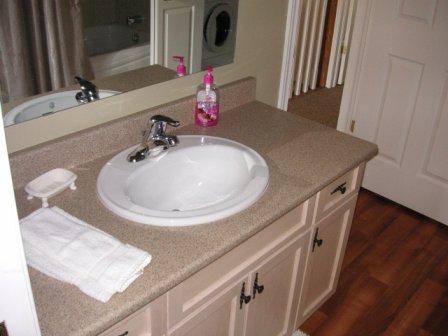The image showcases a bathroom interior captured at an angle, with the sink area prominently displayed on the left and the open doorway on the far right. The door and its frame are both painted white, contributing to a clean and minimalistic aesthetic. The bathroom counter and cabinets have an off-white, beige hue, with the countertop resembling beige granite.

Centrally positioned on the counter is a single white sink, equipped with modern chrome fixtures featuring a single handle that lifts to turn on the water and pushes down to shut it off. To the right of the sink, a bottle of soap with a distinctive pink pump handle and label adds a splash of color. On the opposite side, a porcelain soap dish with raised legs, reminiscent of a miniature doll's bathtub, sits elegantly on the left. Additionally, a neatly folded hand towel lies on the left side of the countertop, ready for use.

Spanning the entire length of the countertop, a large mirror is affixed to the wall, reflecting the bathroom's features and enhancing the sense of space within the room.